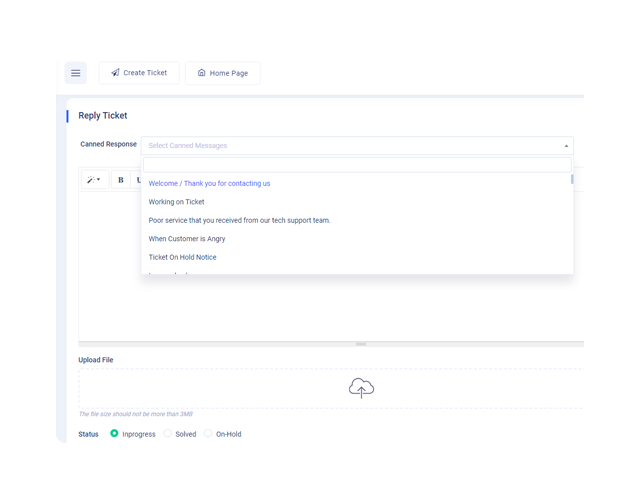A detailed and cleaned-up caption for the image would be:

"The image depicts a user interface with a predominantly white background. In the top left corner, there's a hamburger menu featuring two options: 'Free Ticket' and 'Home Page.' Below this menu, a white box contains the main content. At the top of this box, there's a flyer ticket icon followed by the label 'Correct Response.' Adjacent to this is a long rectangular search bar that displays a drop-down menu when clicked, offering several preset responses such as 'Welcome,' 'Thank you for contacting us,' 'Working on ticket,' 'Poor service received from our support team,' 'When a customer is angry,' 'Ticket on,' and 'Head notice.'

Further down, there is an empty space followed by another box containing a 'Boom File' option along with an upload feature symbolized by the Google Cloud icon positioned centrally. Finally, at the bottom of the interface, a menu allows the user to set the status of a ticket with options including 'In Progress,' 'Solved,' and 'On Hold.'"